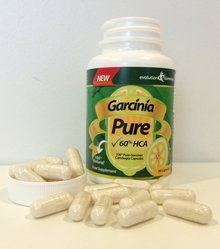The image is a small, low-resolution, color photograph in portrait orientation, depicting a white plastic bottle of pills with its cap removed and placed upside down to the bottom left of it. The focus of the image is on the bottle and the scattered pills on a cream-colored surface. The cap is filled with more of the light brown, shiny pills, some of which have also spilled out in front of the bottle. The label on the bottle features the brand name "Garcinia" with "PURE" prominently written underneath, accompanied by a green tick mark. Below, it states "60%" with the letters "HCA" in capital letters, indicating the content of the supplement. There is also an illustration of a lemon cross-section, suggesting a possible lemon flavor. The label background is green with some red, yellow, and dark green elements, and the word "NEW" appears in white on a red background at the top left corner of the sticker. Some text is hard to read due to the low resolution and parts not being in English.